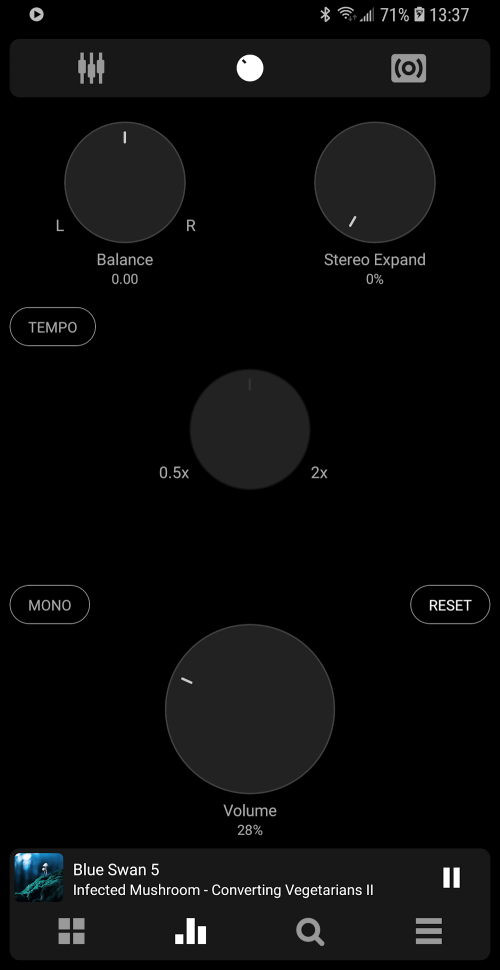This vertical image, typically viewed on a smartphone, features a predominantly black background, devoid of any texture or dimension, creating a solid one-dimensional appearance. 

In the upper left corner, there is a small gray circle with a black triangle, resembling a play button. Opposite, in the upper right corner, are several standard status icons: Bluetooth, Wi-Fi, signal bar strength, and battery life at 71%. The time displayed in military format is 13:37.

Beneath this, a dark gray strip runs horizontally across the screen. On the left side of the strip, various plugin icons are visible, while the center features a white circle with a black dot, resembling a camera icon. 

Further down, in the main section, there are several gray circles with different labels and indicators:
- The first circle, labeled "Balance," shows 'L' and 'R' on either side with a top line, indicating a balance of 0.
- The next circle indicates stereo expansion, marked with a line towards the bottom, set at 0%.
- Another circle displays tempo, with a surrounding bar, marked at 0.5X to 2X. There are additional options for mono, reset, and volume, set at 28%.

The bottom of the image includes text displaying "Blue Swan," "Infected Mushroom," and "Converting Vegetarians." Along with these, there are various icons available for selection.